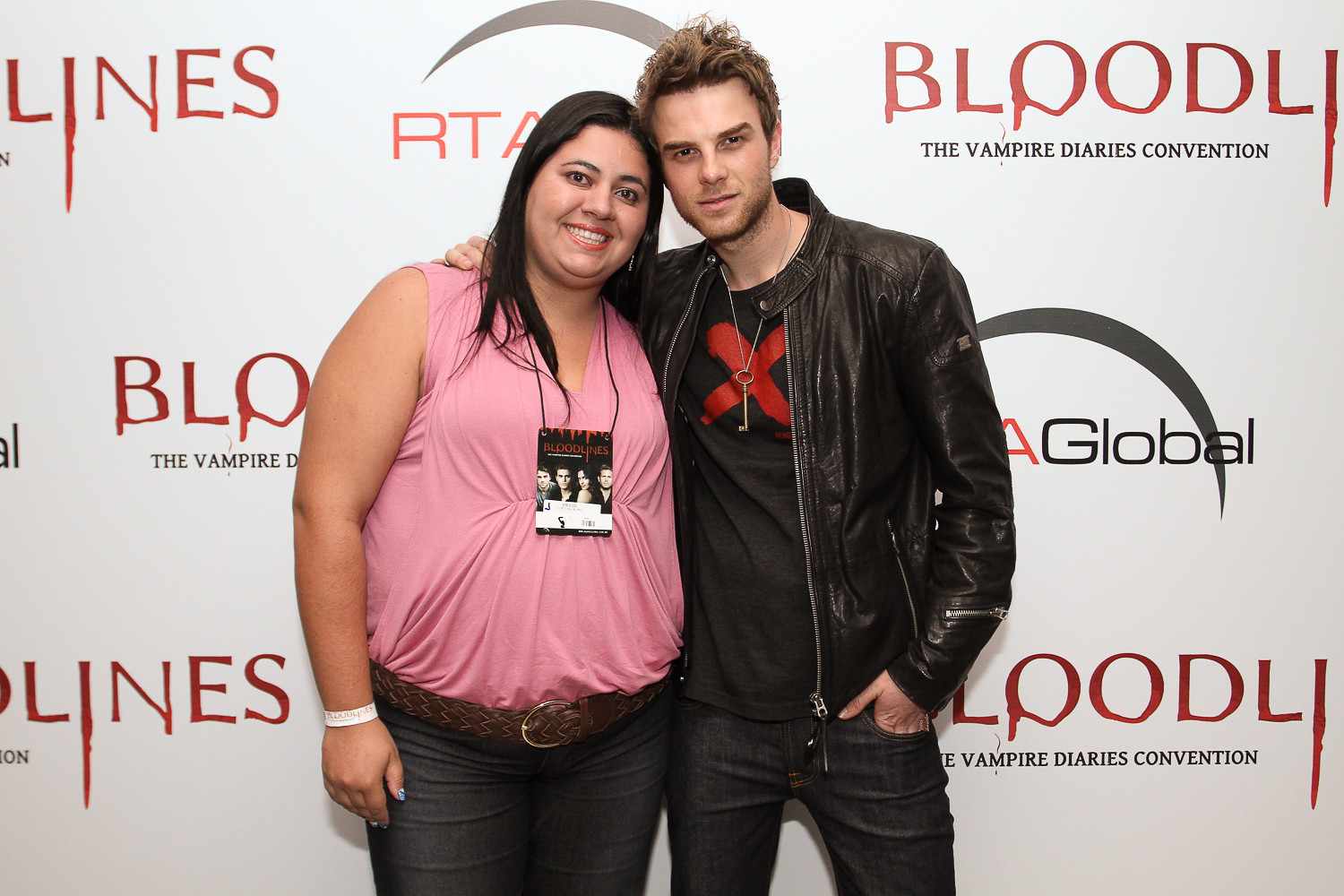In an indoor photograph slightly wider than it is tall, two individuals are captured standing in front of a light gray wall adorned with repeating logos and text. The logos feature the words "Bloodlines" in red, with "The Vampire Diaries Convention" in black underneath. Another logo, reading "RTA Global" with the letters "RTA" in red and "Global" in black, is also visible. The background text includes elements resembling dripping blood on some of the letters in "Bloodlines."

On the left side of the image stands a woman with light brown skin and straight dark brown hair, who appears slightly heavier set. She is dressed in a pink sleeveless top that cinches in the center, a brown leather belt, and dark blue jeans. Around her neck, she wears a lanyard with a picture featuring four cast members from the TV show "The Vampire Diaries." She sports a somewhat awkward smile, has a white bracelet on her wrist, and her nails are painted blue.

To her right, with his arm casually draped around her shoulders, stands a man of Caucasian descent with messy short brown hair and a slight five o’clock shadow. He wears a long-sleeve black leather jacket, open to reveal a black T-shirt with a large red "X" on it. A key hangs from a chain around his neck, and he wears blue jeans. His expression is rather serious, contributing to the overall awkwardness of the pose.